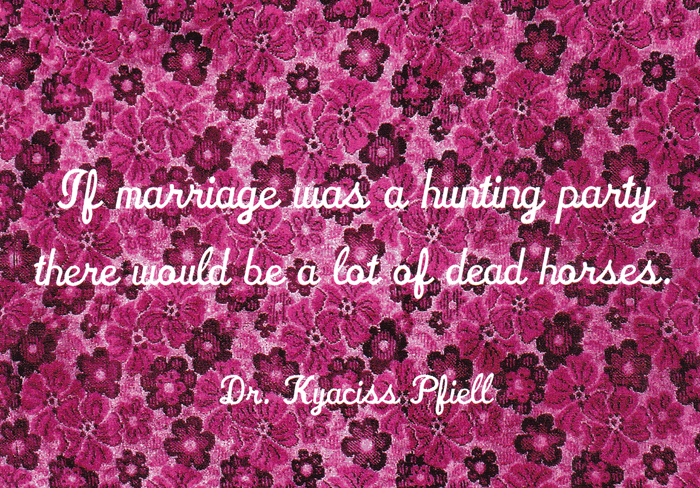The image is a graphic featuring an inspirational quote set against a richly textured floral background. The backdrop consists of a repeating pattern of intricate pink and burgundy flowers, designed to resemble a needlepoint canvas or fabric. Over this floral tapestry, a quote in elegant, white cursive font declares, "If marriage was a hunting party, there would be a lot of dead horses." This poignant message is attributed to Dr. Kyassis Pfiel, with the name spelled K-Y-A-C-I-S-S P-F-I-E-L-L. The cohesive design of the image, combined with the floral motif and the delicate cursive script, creates a visually appealing and thought-provoking graphic.